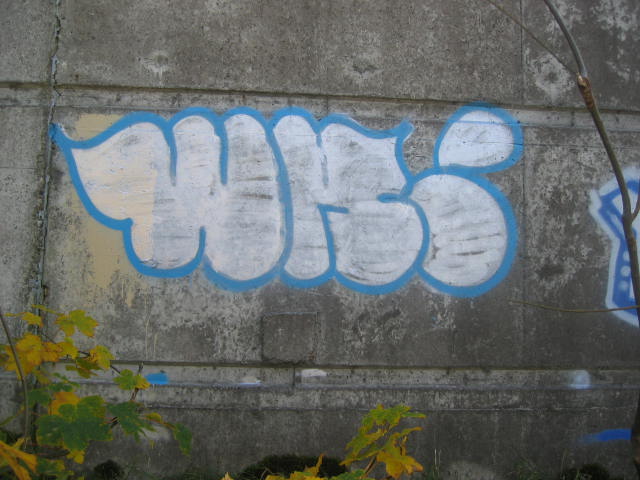The photograph captures an older concrete wall completely filling the frame, adorned with graffiti art. The wall features two horizontal recessed strips – one above and one below the graffiti. Positioned about five feet from the wall, the camera provides an unobstructed and intimate view of the artwork. The graffiti, composed of three vibrant and playful words, appears in a standard graffiti style with white letters accented with light blue borders. The white paint, potentially chalk-based due to its somewhat transparent appearance, stands out against the weathered gray concrete. The letters W-H-O are distinct, though the ‘O’ has an unusual accent, perhaps making it look like the word ends with an extra flourish or a period. 

Embedded within a section resembling a rectangular slab, the graffiti is framed by the rough textures of the aged concrete. Below the wall, at the bottom edge of the image, there's yellowing vegetation – a couple of plants, one in the bottom left corner and another near the center, both exhibiting brown and green leaves indicative of autumn. These plants, extending slightly into the photo, further emphasize the wall’s longstanding presence by suggesting it stands behind a set of untended bushes.